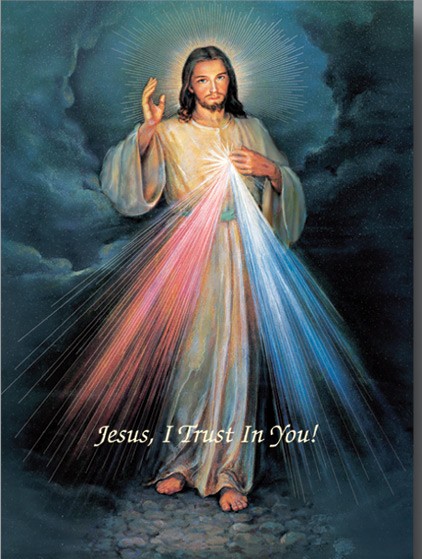This vertically aligned rectangular image resembles a greeting card and portrays Jesus Christ. Jesus is depicted with long hair, a beard, and a white robe, standing barefoot on rocky ground. He has his right hand raised and his left hand touching his heart. Emerging from his heart are two beams of light: a pink one on the left and a blue one on the right. A radiant light halo surrounds his head, sending out various rays. There are blue and gray clouds in the background, with darker shades on the upper right side. At the bottom of the image, across Jesus' shins, the text "Jesus, I trust in you!" is written in white.